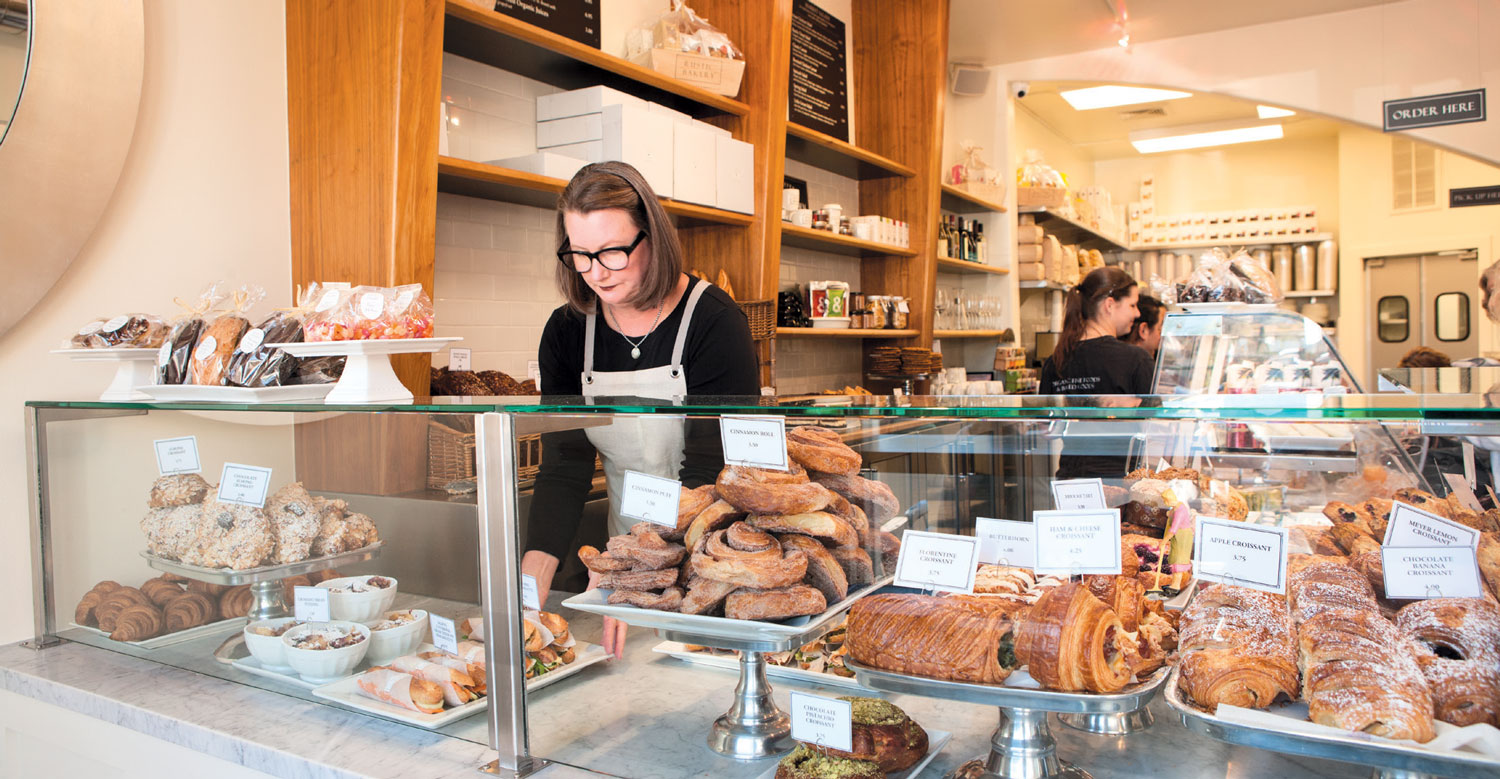In the bustling interior of a small bakery, a prominent glass-fronted countertop displays an array of tantalizing pastries on silver trays, some flat and some raised on stands. Behind this glass partition, there are cinnamon rolls, doughnuts, and bread stuffed with chocolate and dusted with powdered sugar. To the left on the countertop, there are some packaged items ready for sale. Behind the counter, a woman dressed in a white apron over a long-sleeved black shirt meticulously adjusts a tray. She has short brown hair, black-framed glasses, black lipstick, and a silver necklace with a pendant. The scene is lively with another female worker visible further inside the store, attending to other trays beneath additional glass counters. The shop is well-lit, with shelves full of products visible beyond the counter, and signs hanging from the ceiling indicating areas for ordering and picking up.